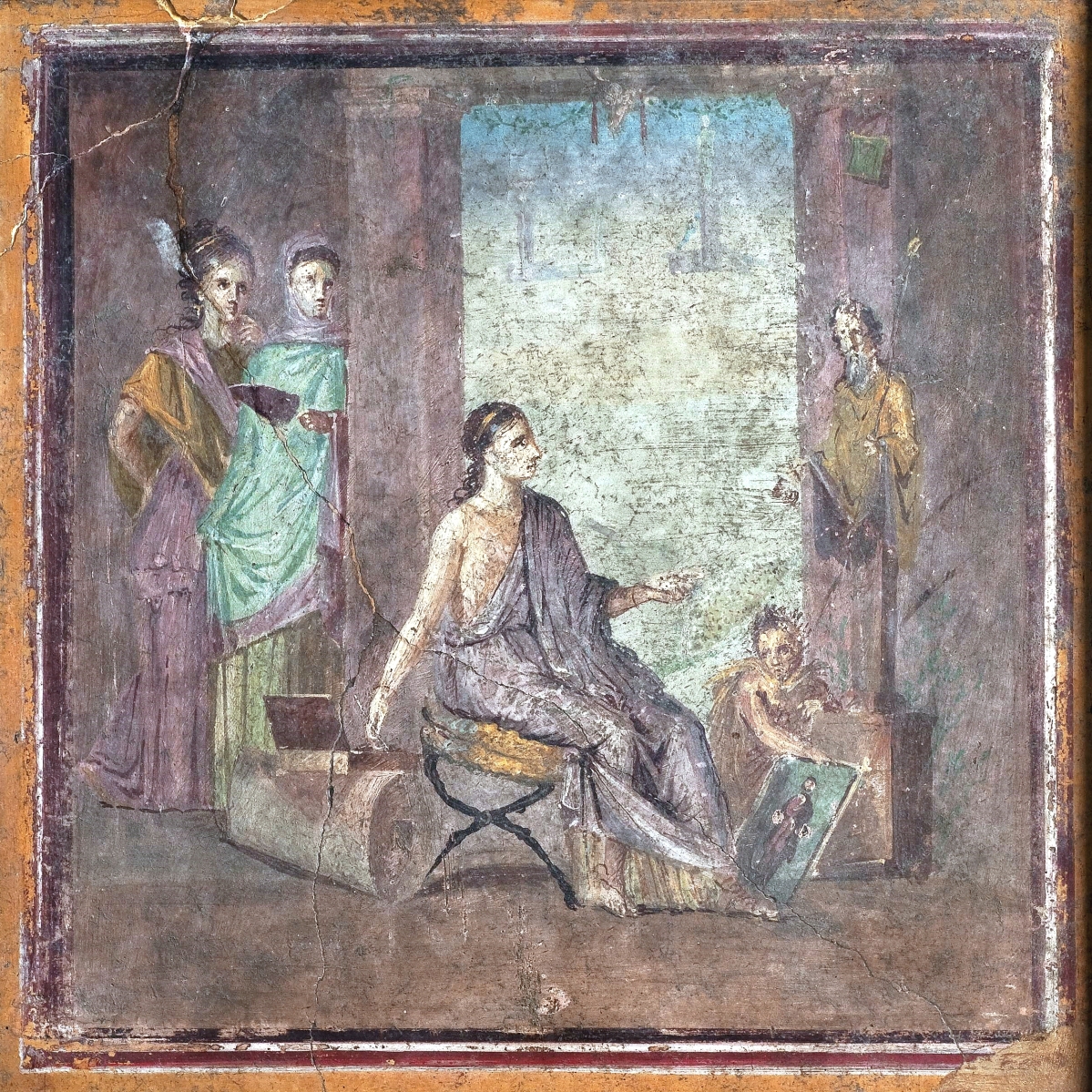This is a weathered and cracked square painting with a wooden, brown frame, portraying an intriguing indoor scene. Dominating the center of the painting is a person seated on a stool or chair, wearing a one-shoulder robe tied at the waist, with hair styled in a low ponytail. In front of this central figure hovers a very slender man, adding a surreal element to the composition. By the doorway, two women are dressed in strikingly colored attire—one in a green dress with a sash and her hair styled half up and half down, and the other in a purple and blue long dress with a headscarf, appearing to watch the scene unfold. A child near the right side seems to be holding a photograph or small painting, and nearby, an elder gentleman gazes intently at the central figure. The doorway depicted opens to an exterior awash in green hues, with large pillars framing the scene. The painting, once vibrant with colors like teal, yellow, lilac, browns, and reds, now appears faded and dull due to extensive wear and tear, with pronounced cracks and worn-off paint. The frame, detailed with purple, red, and black, bears testament to its age.